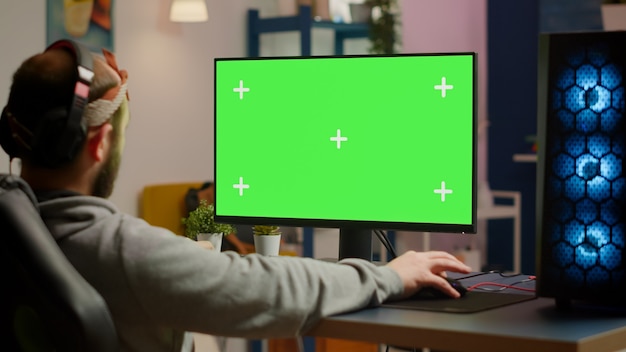In this color photograph, a young man sits in a cushioned black gaming chair at a brown desk, engrossed in a computer monitor displaying a fluorescent green screen with five white crosses—one in each corner and one in the center. He is in a three-quarter pose, his right hand on a computer mouse, partially away from the camera, revealing his right ear and short brown beard. The man, who is wearing a gray sweatshirt and a reddish cap, has his headphones placed off one ear. A tall black piece of equipment with three blue lights, likely a speaker, stands to his right. Behind the monitor on the left, there are two white ceramic pots with green plants. The background is slightly out of focus, hinting at a room with possibly a chair and blue shelving, but the details remain unclear.